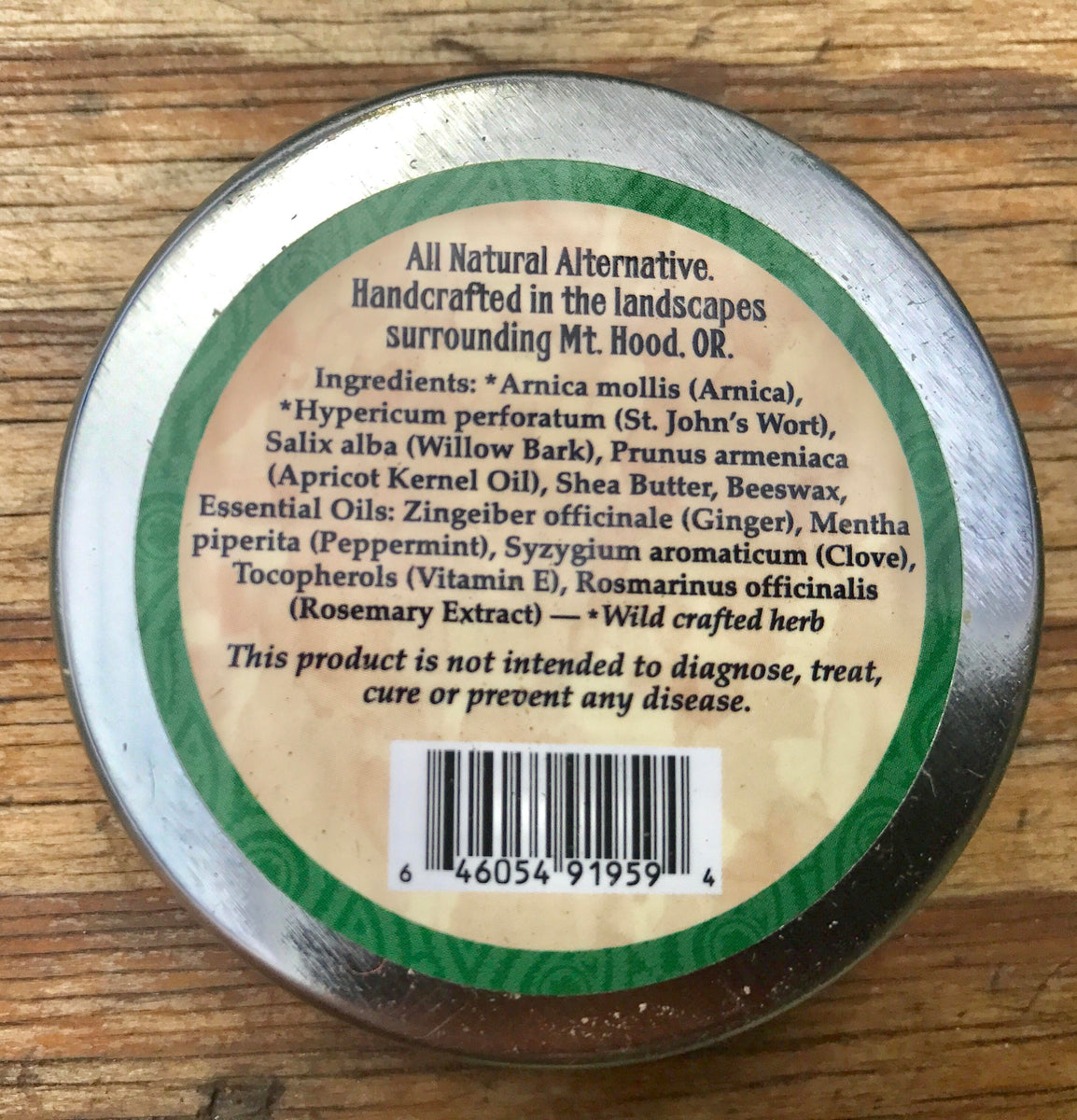The image captures a close-up photograph of the bottom of a round, silver-toned metal can, positioned on a wooden surface with varying shades from beige to dark brown and subtle signs of peeling paint. The can features a circular label with a green border and a light brown, almost tan background. Prominently displayed at the top of the label in black text are the words: "All Natural Alternative, Handcrafted in the Landscapes Surrounding Mt. Hood, Oregon." Below this, the label presents a detailed list of ingredients, followed by a disclaimer stating, "This product is not intended to diagnose, treat, cure, or prevent any disease." At the bottom of the label, there is a black barcode. The can itself shows minor scratches and chips, with a few white grains of sediment visible towards its base.